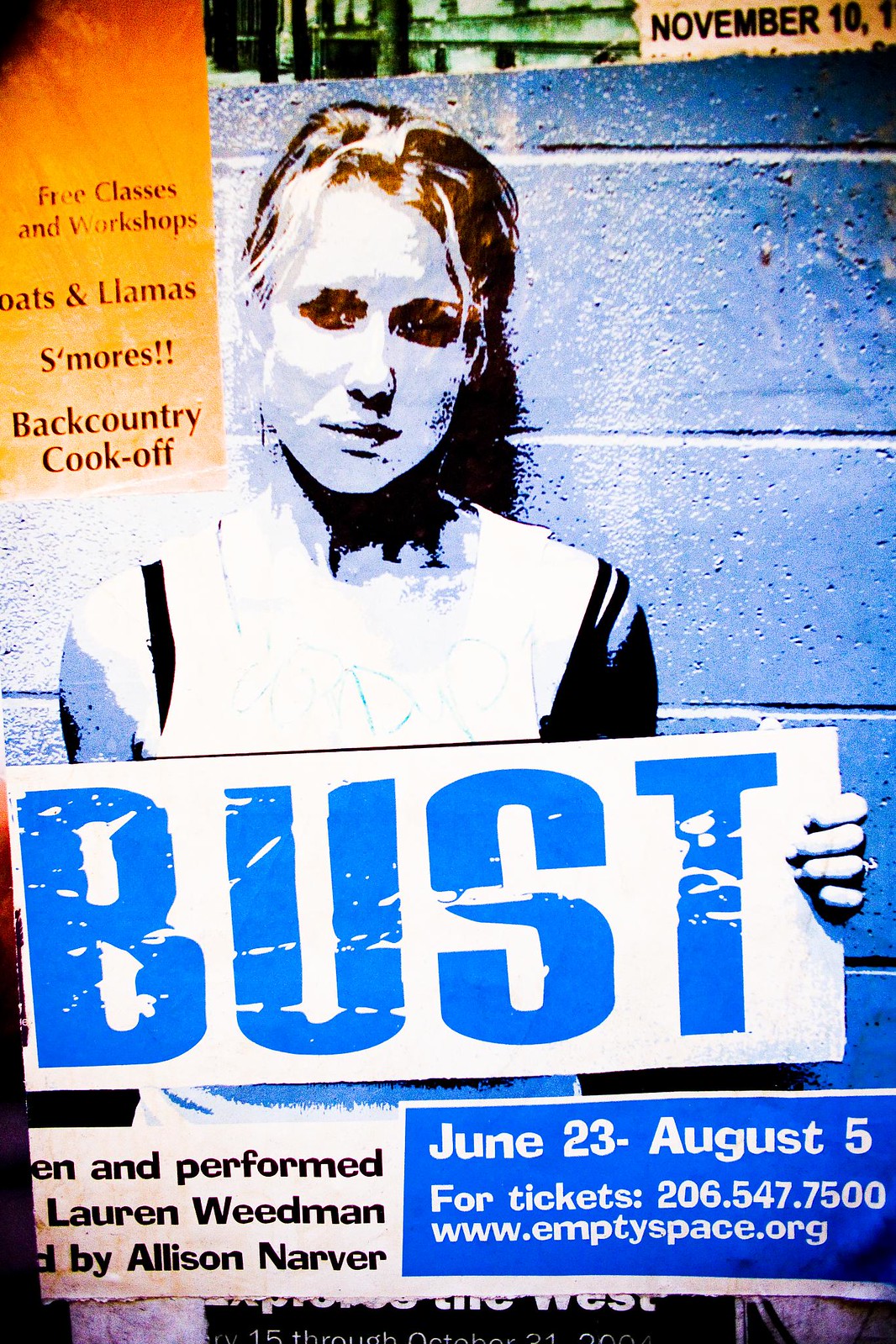The image features a vibrant, multicolored poster for an upcoming theatrical play titled "BUST." At the center of the poster stands a stylized image of a woman with predominantly white and brown hair, her face painted white. She holds a sign with bold blue letters that spell "BUST." The background behind her is a blue brick wall. Below the sign, additional text provides details about the play: "An Unperformed Lauren Weidman by Allison Narver," and the performance dates, "June 23rd - August 5th." There is also a phone number and a website for tickets: www.emptyspace.org.

In the top right corner, an orange box contains the text "FREE CLASSES AND WORKSHOPS, BOATS AND LLAMAS, S'MORES, BACKCOUNTRY COOK-OFF." This same information is repeated in a blue box on the bottom right corner. The poster features a varied color palette, including black, orange, yellow, white, blue, pink, purple, and green. The overall design gives the impression of a lively and engaging advertisement for a theatrical event.